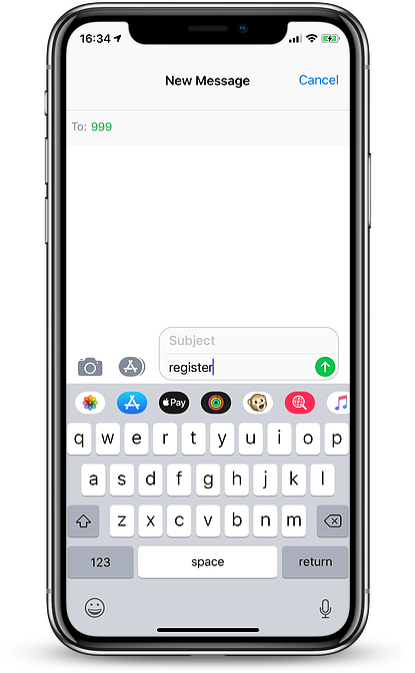The image portrays a smartphone with a black frame set against a white background, casting a subtle drop shadow below it. The device's screen is illuminated, displaying a mobile user interface. 

In the status bar at the top, the current time is shown as "16:34" on the left side, accompanied by a location icon. On the right side, there are three out of four cellular signal bars, a fully connected Wi-Fi icon, and a battery indicator showing it is charging, represented by a horizontal battery outline filled with green and a black lightning bolt symbol. This status bar is set against a light gray background.

Dominating the center of the screen, there's a notification area with "New Message" written in bold black letters. To its right, "Cancel" is displayed in blue. Below this section, there's a thin gray line separating the "To:" field, which contains the numbers "999" in green, hinting at an emergency contact or placeholder number.

Beneath the recipient's section is the blank message composition area, which is entirely white and currently empty. The user appears to be in the process of typing a message.

At the bottom, the iPhone's keyboard is visible. To the left above the keyboard, dark gray icons for the camera and a unique bone-like symbol are located. Below these, there's a light grey outlined rectangle with "Subject" written in it, and underlined text that reads "register" in lowercase. Adjacent to this text is a green circle featuring a white upward-pointing arrow.

Above the keyboard, several icons are aligned, including:
1. A photo icon.
2. An "A" inside a blue oval.
3. An Apple Pay icon.
4. A target-like symbol inside a black circle.
5. A small brown monkey housed within a white oval.
6. A search icon atop a vibrant red-pink background.
7. An Apple iTunes icon.

The keyboard itself follows the standard QWERTY layout, with rows of alphabetical characters. Icons for an emoji keyboard and a microphone are found at the bottom left and the bottom right corners respectively. The bottom row includes essential keys like space, numeric toggle ("123"), and return.